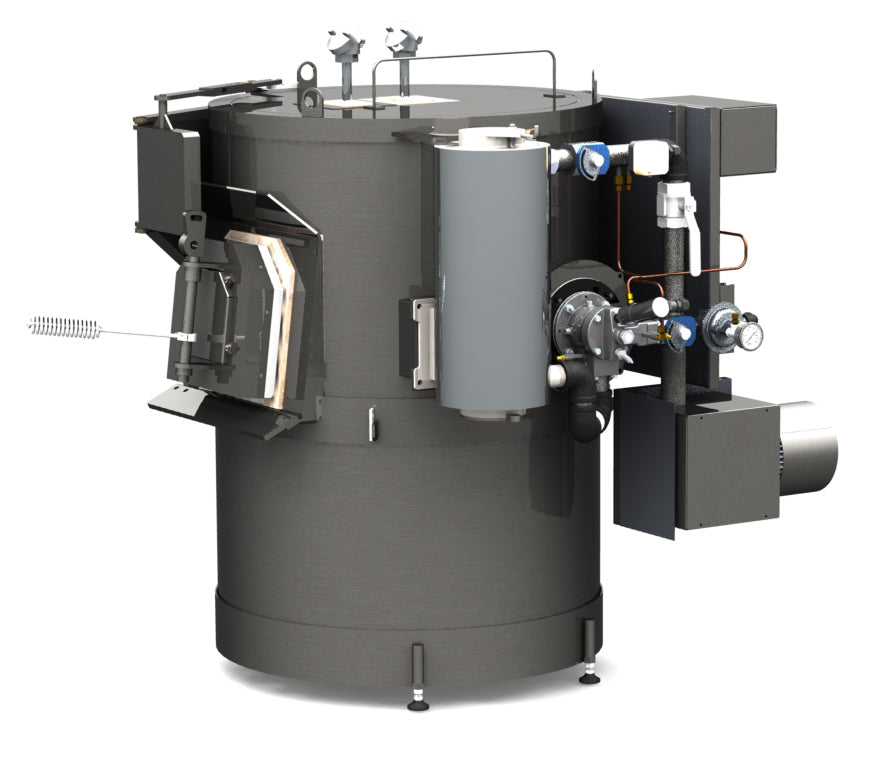The image showcases a detailed photograph of a large, dark gray industrial cylindrical device standing vertically, resembling a combination of a water heater and a pumping or heating mechanism. The main cylinder serves as the core structure, complemented by an array of intricate attachments and components. A smaller, lighter gray cylinder is affixed slightly towards the upper right section of the main cylinder, along with various rectangular and circular contraptions projecting outward. 

On the right side, an attachment extends from the upper part, featuring rods that connect to a square bottom portion with a pipe-like extension. The left side of the machine bears a unique five-sided steel plate with an antenna-like structure emerging from its center. Additionally, the top is marked by a network of valves, pipes, and blue and white dials, contributing to its complex appearance. The device is supported by small, black and white feet positioned at the bottom, suggesting a somewhat unsteady balance. All these elements are set against a stark white background, further emphasizing the intricacy and mysterious functionality of this heavy-duty industrial apparatus.